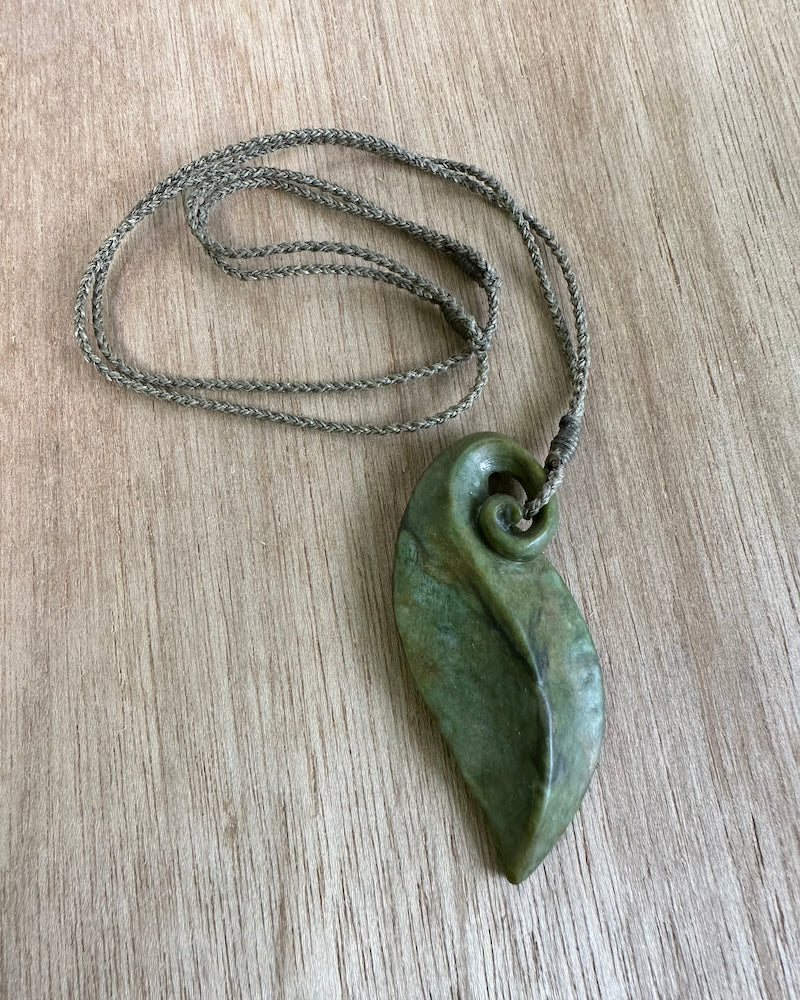This photorealistic image captures a unique necklace resting on a piece of light-colored, grayish wood with vertical grain patterns. The necklace features a thin, braided nylon rope that curls into a loop above the pendant. The pendant itself is an abstract gemstone, reminiscent of jade, with a faded sea green hue that evokes the natural beauty of a leaf or a curved arrowhead. This gemstone has a striking 3D shape, with the top twisting and twirling to create an eye hole where the rope is attached. The design is further detailed by a central ridge that adds depth and texture, accentuating the gem's leaf-like or S-shaped structure.